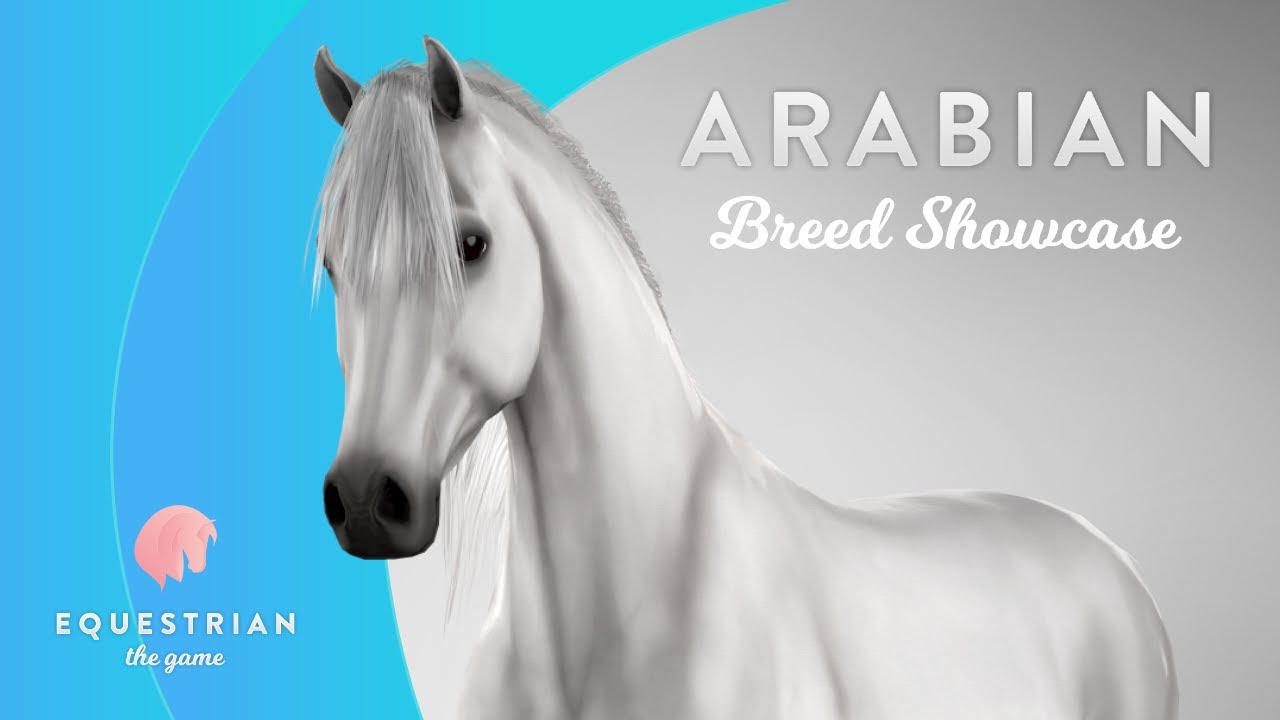The image appears to be an advertisement featuring an illustrated or computer-generated white and gray horse with a black snout and black-inside ears. The horse's mane is short, and its body is angled slightly to the right with the face almost forward, giving prominence to its dark eyes. The background includes a blend of blue and aqua curves on the left side, transitioning into a silvery gray area, and features a pink horse head icon. The top right corner of the image displays the words "Arabian Breed Showcase" in white text, with 'Arabian' in capital letters and 'Breed Showcase' in cursive. In the lower left corner, written above the pink horse head, are the words "Equestrian The Game," with "Equestrian" in capital letters and "The Game" in cursive. The image cuts off just past the horse's chest, not showing its legs.